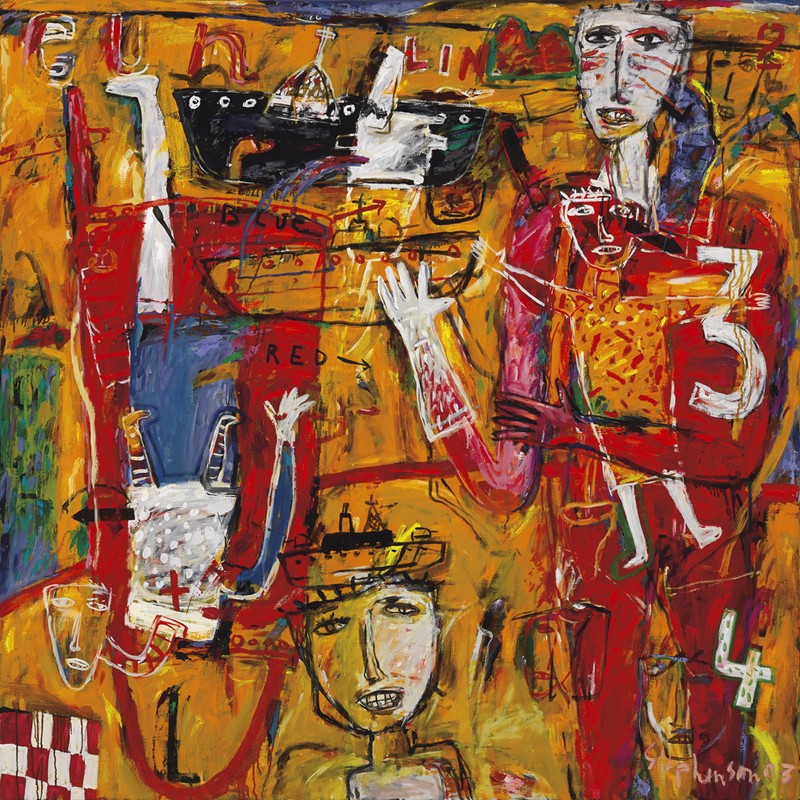The image is a vibrant and intricate modern art painting with a whimsical, somewhat cluttered style, reminiscent of works from the last 20 years. The main background is a vivid blend of yellow shades, interspersed with various other colors like reds, blues, and greens. Central to the image are three distinct human figures, with one more prominent on the right side, dressed in red pants and a long-sleeved shirt, marked with the number "3" in white on the torso. This main figure has a white neck, a face with sincere, slightly smiling eyes, short hair, and a long nose, giving an impression of a male. 

Overlaying this figure is a smaller body with disproportionately large shoulders and simple limbs, which seems to be facing the main figure. This smaller body has an orange hue and is capped with a witch-like head.

Towards the center-left, there's an upside-down figure wearing a white shirt with a red "X" and possibly blue shorts, featuring an extended white arm with the word "RED" above their hand. This figure has a long, white neck and a mask-like face, with only one foot visible, contributing to the surreal composition. 

Additional elements include a blue background interwoven at the bottom left, a face sketched in black with the yellow background showing through, and various objects, including ships and an animal head possibly resembling a smiling sheep. Letters and numbers like "EU," "N," "3," and "4" are scattered across the painting.

Amidst the rich tapestry of colors and forms, the painting captures a sense of playful chaos, with red checkerboards, blue crosses, and intricate, overlapping textures that evoke a feeling of both spontaneity and deliberateness.